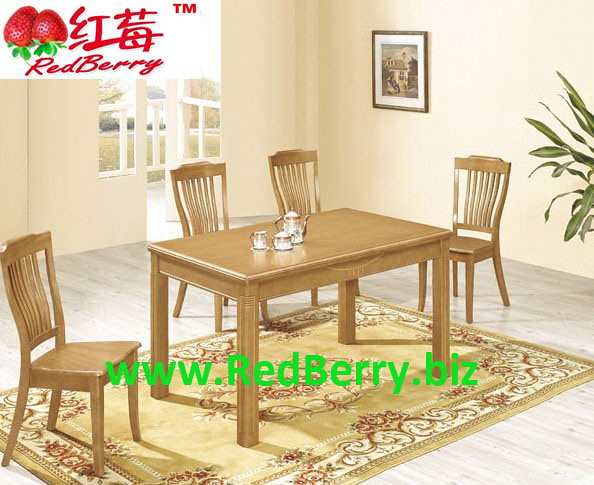This image is a photograph likely designed for an online retailer or catalog advertisement, showcasing a dining room set by the brand Redberry. The dining area features a light brown wooden table positioned centrally in the image, flanked by four matching wooden chairs—one at each end and two along the longer side, all facing the camera. The table itself has simple, rectangular contours with a slight carved design on its legs, adding a touch of elegance to its otherwise minimalist appearance.

On top of the table is a small tea set, including a silver teapot and two matching teacups, giving a cozy, inviting touch to the scene. The dining set rests on a Persian-style rug, predominantly green and brown, which complements the wooden furniture. White walls surround the setup, adorned with a framed photograph, and a door is visible behind the table, slightly ajar.

Branding elements are prominently displayed within the image. In the top left corner is the Redberry logo, featuring two inverted red strawberries alongside Asian characters, and below them, the brand name is written in a pseudo-cursive red font with a small trademark symbol. Across the middle of the photograph, the website URL, "www.redberry.biz," is displayed in a vibrant neon green font, ensuring brand visibility.